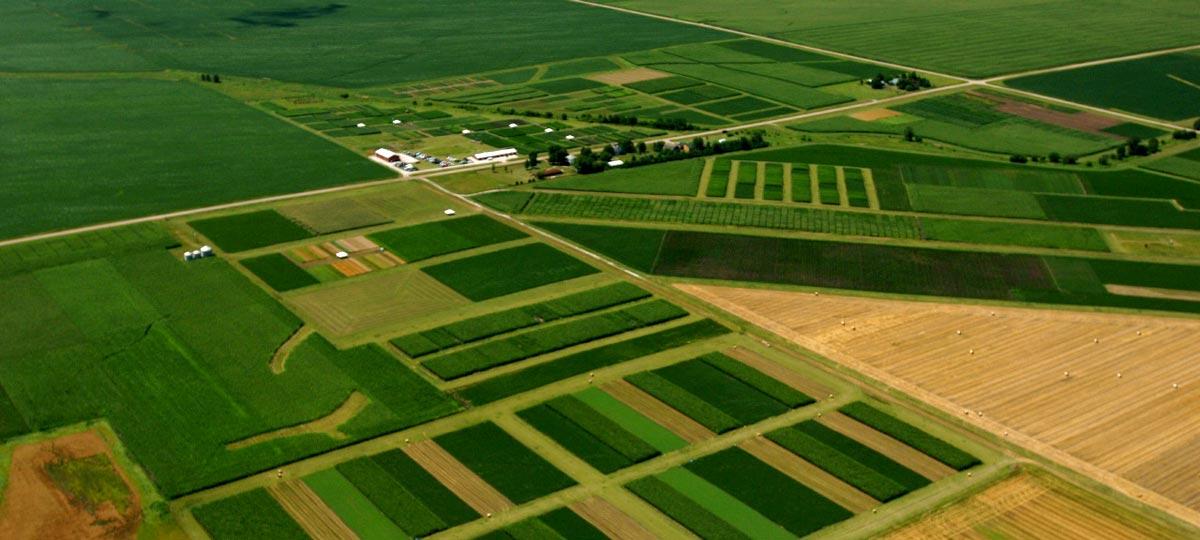This aerial photograph showcases an expansive agricultural landscape divided into various geometric plots. The majority of the farmland consists of several large rectangular fields, approximately seven in total, which are predominantly green with varying shades, indicating diverse crops. The fields are meticulously plowed, exhibiting clear rows of vegetation. In the lower foreground, there's a distinct contrast with bands of deeper and lighter greens, and a noticeable tan-colored triangular area, suggesting prepared but unplanted soil.

A paved road cuts diagonally across the farmland from the middle left to the upper right quadrant, intersecting at a crossroads where a few trees and white, roofed structures—likely houses or farm buildings—are situated. From the lower right corner, another road converges towards the crossroads, enhancing the organized layout of this agricultural area. This detailed aerial view not only encapsulates the structured and varied nature of farmland but also highlights the intricate patterns and shades of green that define a thriving agricultural landscape.